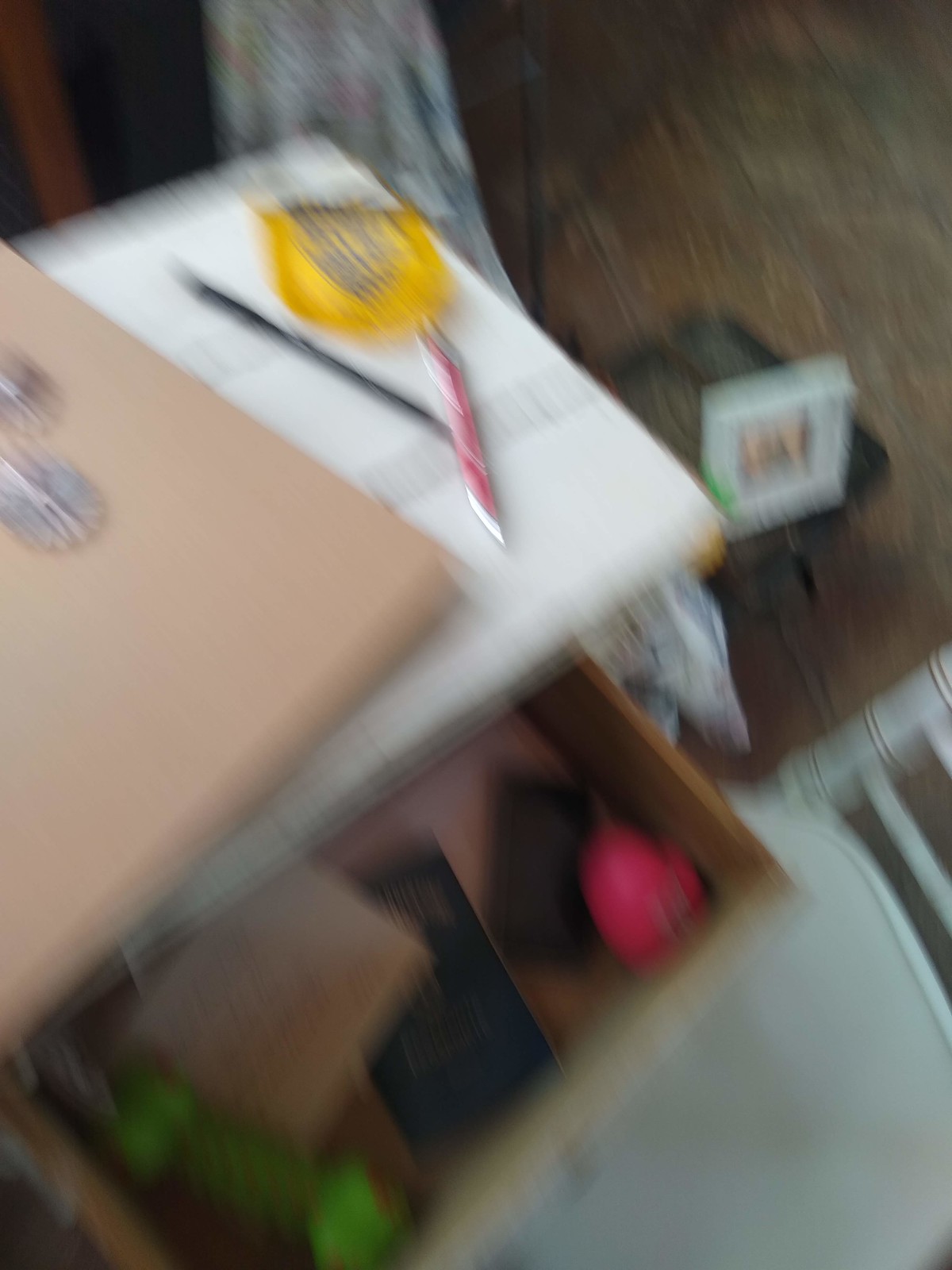In this slightly blurry photograph, we see a small, white end table with an open drawer. Inside the drawer, various items are visible, including a cell phone, a red ball, and a green object situated in the left corner. The end table’s surface features a few gray stripes and partially supports a tan laptop cover adorned with a sticker. Atop the table rests a circular yellow item, a red and silver stick-like item, and what seems to be a black pen. In the lower right corner of the image, a white, wooden chair is partially visible. To the right of the chair stands a small black table with black legs, on which a white-framed picture displaying two faces is placed. Behind this setup, a white and blue curtain extends from the mid-left of the frame to underneath the corner of the small table on the right side.